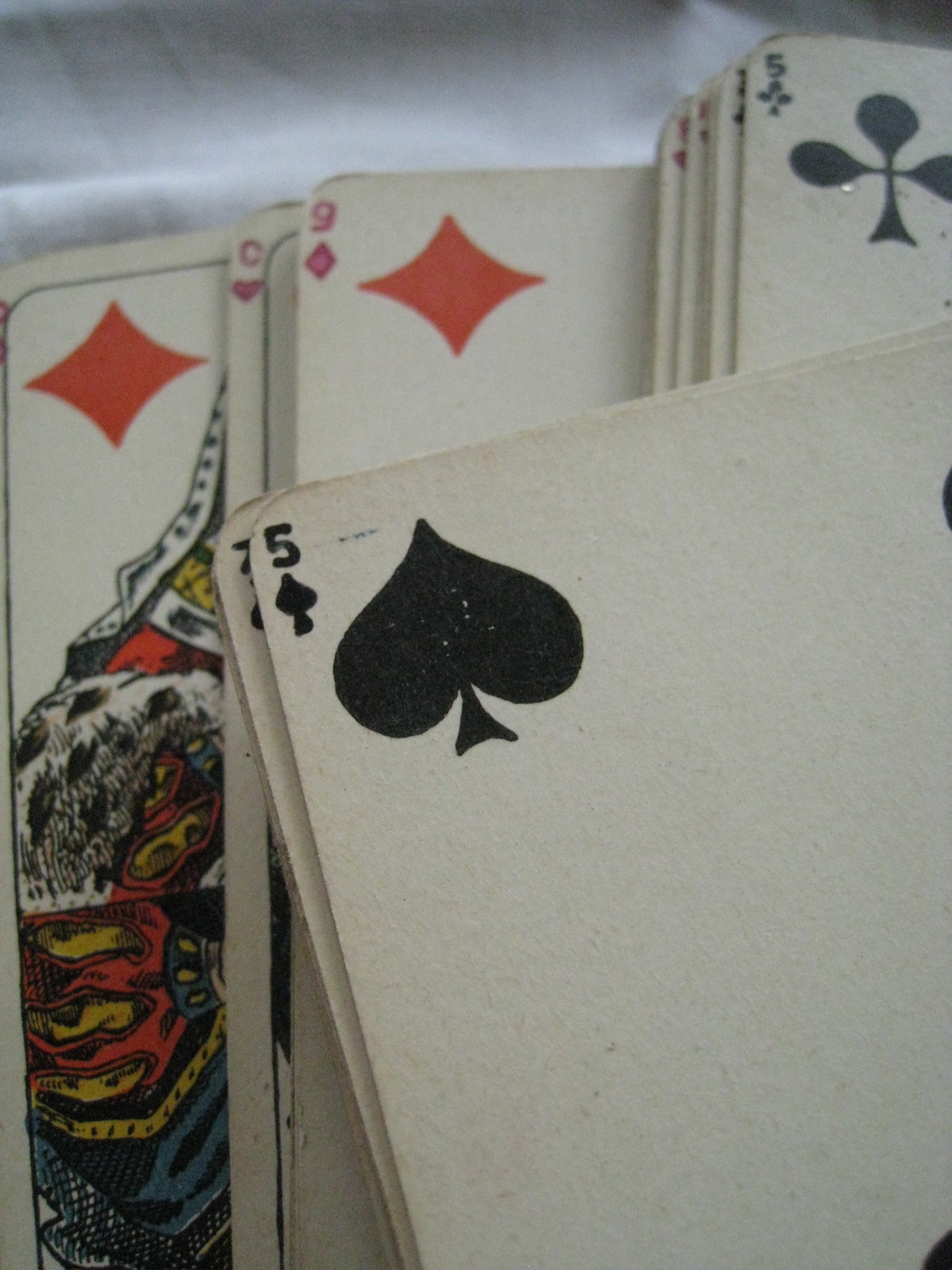This photo features a stack of well-worn playing cards arranged in a portrait orientation. The cards are layered such that some fully obscure the ones beneath them while others allow partial glimpses of the cards below. The prominent card in the image is the Five of Spades, positioned towards the center, displaying a small spade symbol and the numeral '5' in the upper left corner, with a larger spade directly beneath it. The card is largely blank aside from these markings, with hints of two more spade logos peeking from the upper and lower right corners.

Behind the Five of Spades, the corners of other cards create a layered mosaic. A partially visible Seven of Spades reveals its black spade symbol. In the lower right-hand corner, another Five of Spades appears in a similar configuration to the central card. Faint colors of underlying cards are perceptible, showing a mix of blacks and reds.

Beneath these, a partially hidden Nine of Diamonds displays the customary red diamond symbols. A Queen of Hearts follows, adding a touch of regal flair with the bold red heart iconography. The bottom card, another member of the diamond suit, presents what appears to be a court card—potentially a Queen, King, or Jack, identified by the visible edges of its intricate illustration.

The background is softly blurred and features a wavy texture that suggests a sheet or fabric, enhancing the vintage aesthetic of the scene. The overall composition captures the nostalgic, timeworn essence of these playing cards, set against a serene and almost ethereal backdrop.